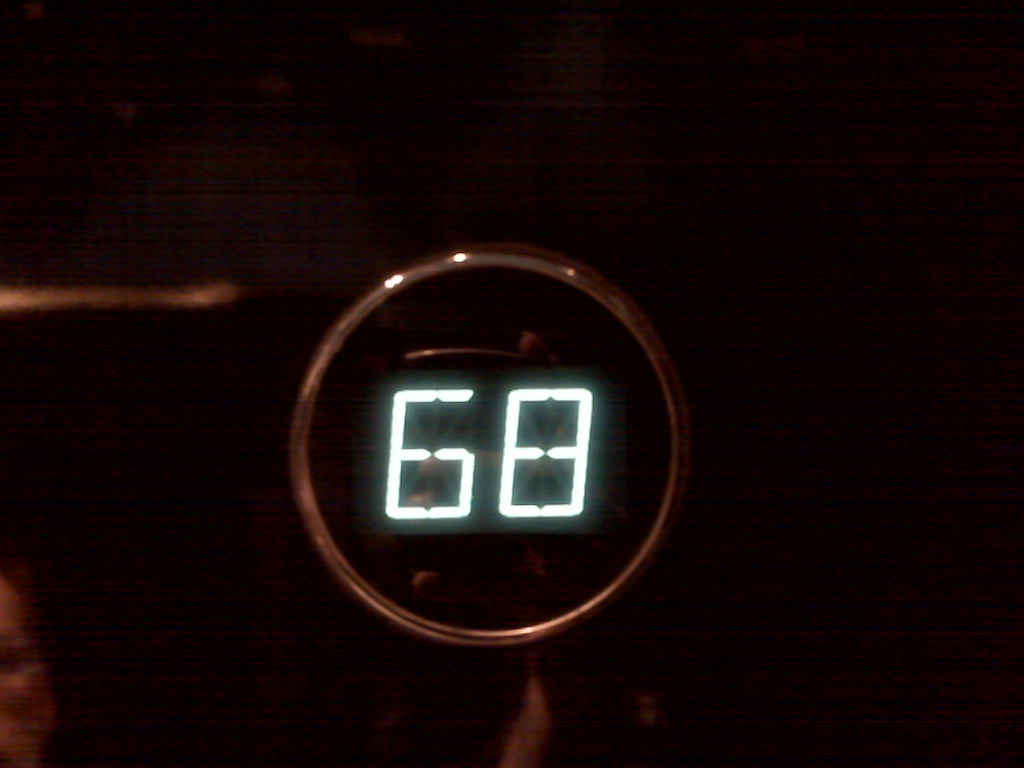The image is set against a very dark background, making it challenging to discern its overall context. Dominating the scene, on the center-left side, there is a lighter brown line extending about a quarter of the way into the image from the left. At the exact center, a circle is visible, rimmed with the same light brown hue. Within this circle, the bright white digital numerals "68" glow prominently. 

Around the 11 o'clock to 12 o'clock positions on the circle's edge, small white dots are visible, likely reflections caused by the radiant white numerals. Just above the digit "6," a faint tan area stretches horizontally from the left side of the "6" to the left side of the "8." Another lighter tan patch is present along the bottom edge of the image, slightly to the right of center, echoing the lighter tones seen elsewhere in the composition.